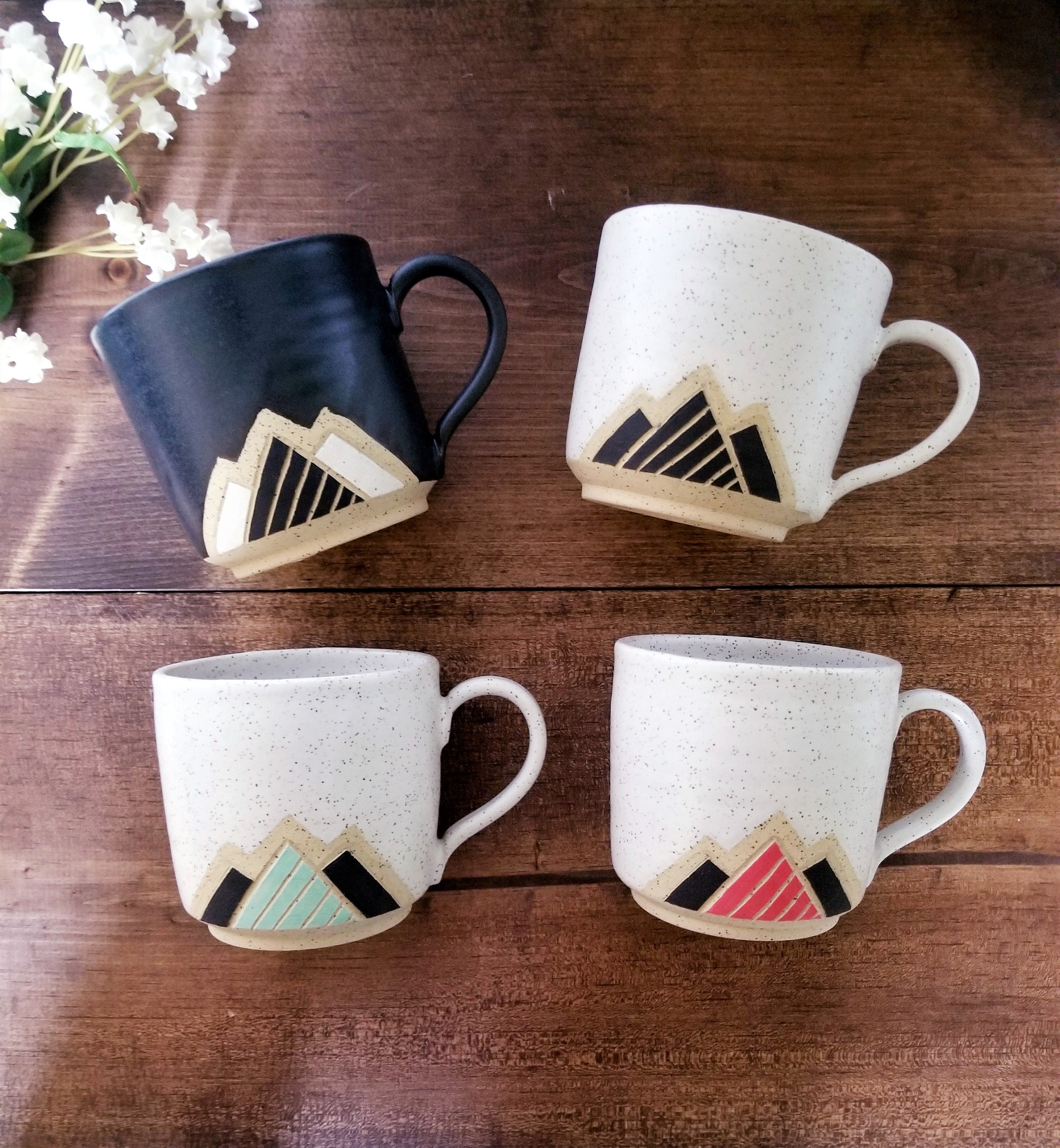The photograph showcases a set of four mugs, arrayed in a neat 2x2 arrangement, all placed on their sides upon a flat, brown wooden surface marked with dark lines. Each mug features a distinctive yet cohesive design, hinting at them being part of a similar set despite their varied colors. The top left mug is black with its handle pointing to the right and is adorned with a pattern of three triangles—two black triangles flanking a single black triangle with intricate black and white markings. The top right mug is white, speckled with gray, and also features three triangles—two black triangles and a central black triangle, marked by lines passing through it. The bottom left and bottom right mugs are white with black dots and possess similar mountain-like designs in beige at their base. These beige mountains display unique color combinations: black and teal on the bottom left mug, and bright pink and black on the bottom right mug. Completing the scene, a bouquet of tiny white flowers on green stems occupies the top left corner, enhancing the cozy, rustic aesthetic of the image.